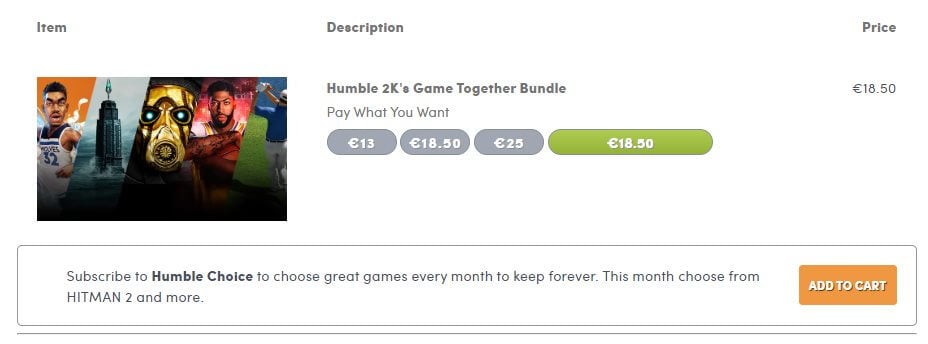This is a screenshot from an unknown website featuring an item menu with columns labeled "Item," "Description," and "Price" at the top. The central image consists of five diagonal slices, each depicting different visuals. From left to right:

1. A cartoon depiction of an African American man wearing a Wolves jersey, numbered 32.
2. A building, encircled at its base by waves.
3. A golden helmet with glowing blue eyes.
4. Another African American man, this time posing with his arms crossed and holding a basketball.
5. A golfer dressed in a blue shirt and white shorts, lifting a golf club over their shoulder.

Below the images, the text reads "Humble 2K’s Game Together Bundle" with a "Pay What You Want" pricing structure. The price options listed are €13, €18.50, and €25, with the user having selected the €18.50 option. 

To the right side, the price of €18.50 is reiterated. Below this, it suggests subscribing to Humble Choice to receive and keep great games every month, highlighting this month's selection, including "Hitman 2 and more."

A prominent orange rectangle, with "Add to Cart" written in white lettering, is displayed at the bottom, inviting users to finalize their purchase.